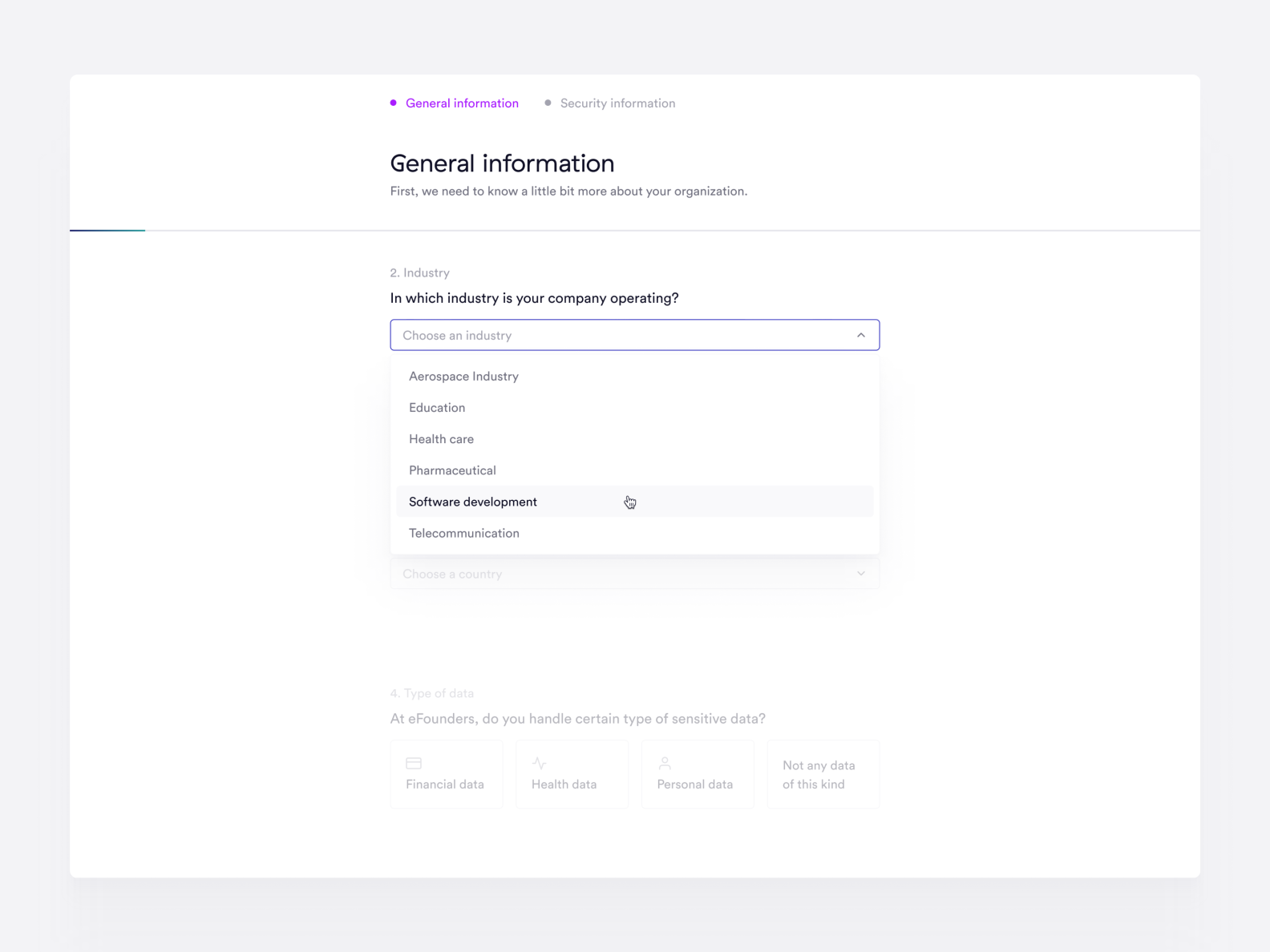The image features a well-structured informational layout. To the left, a purple asterisk appears, accompanied by the text "General Information" also in purple. To its right, a small gray circle marks the section "Security Information." Approximately two inches below this header, "General Information" is prominently displayed in bold black text. 

Following this title, the script explains: "First, we need to know a little bit more about your organization," leading to a long horizontal line. 

Below this line is the numeral "2," with the word "Industry" beside it in light gray. A descriptive question follows in darker text: "In which industry is your company operating?" The options are presented within a long rectangular input box labeled "Choose an industry." Available selections are listed below in black text: Aerospace Industry, Education, Healthcare, Pharmaceutical, and Software Development, while "Telecommunication" is noted in gray.

At the bottom, there is a subtle query in light gray text: "At eFounders, do you handle certain types of sensitive data?"